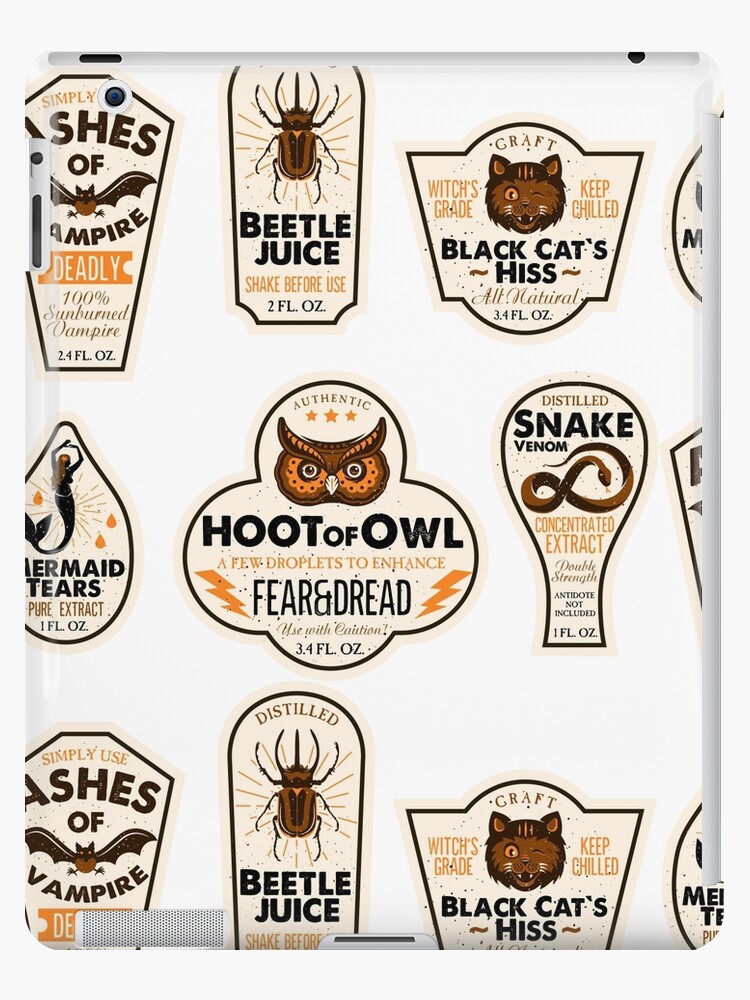In this image, various product labels are displayed against a white background, each featuring an animal illustration and accompanying text. The labels showcase different shapes and sizes, with the animal illustrations predominantly in brown hues. 

On the right, a gray label reads "Craft," featuring the text "Keep Chilled, Black Cat Hiss, All Natural, 3.4 fluid ounces," accompanied by a winking cat image. Adjacent to it, another label with the text "Beetle Juice" instructs "Shake Before Use" and specifies "2 fluid ounces," adorned with a beetle illustration.

Toward the center, a label titled "Ashes of Vampire" marked as "Deadly, 100 Sunburned Vampire, 2.4 fluid ounces" stands out. In the very center, there's a label that reads "Hoot of Owl," which includes the phrase "A few droplets to enhance fear and dread," though part of the text is unclear. This label also indicates "3.4 fluid ounces" and features an owl's face.

To the right of that is a label for "Distilled Snake Venom," described as a "concentrated extract," featuring a snake. Together, these labels create an assortment of fictional products, each illustrated with animals and detailed descriptions. The color palette consists of various shades of browns, beiges, blacks, grays, and some darker hues, enhancing the whimsical and intriguing nature of the image.